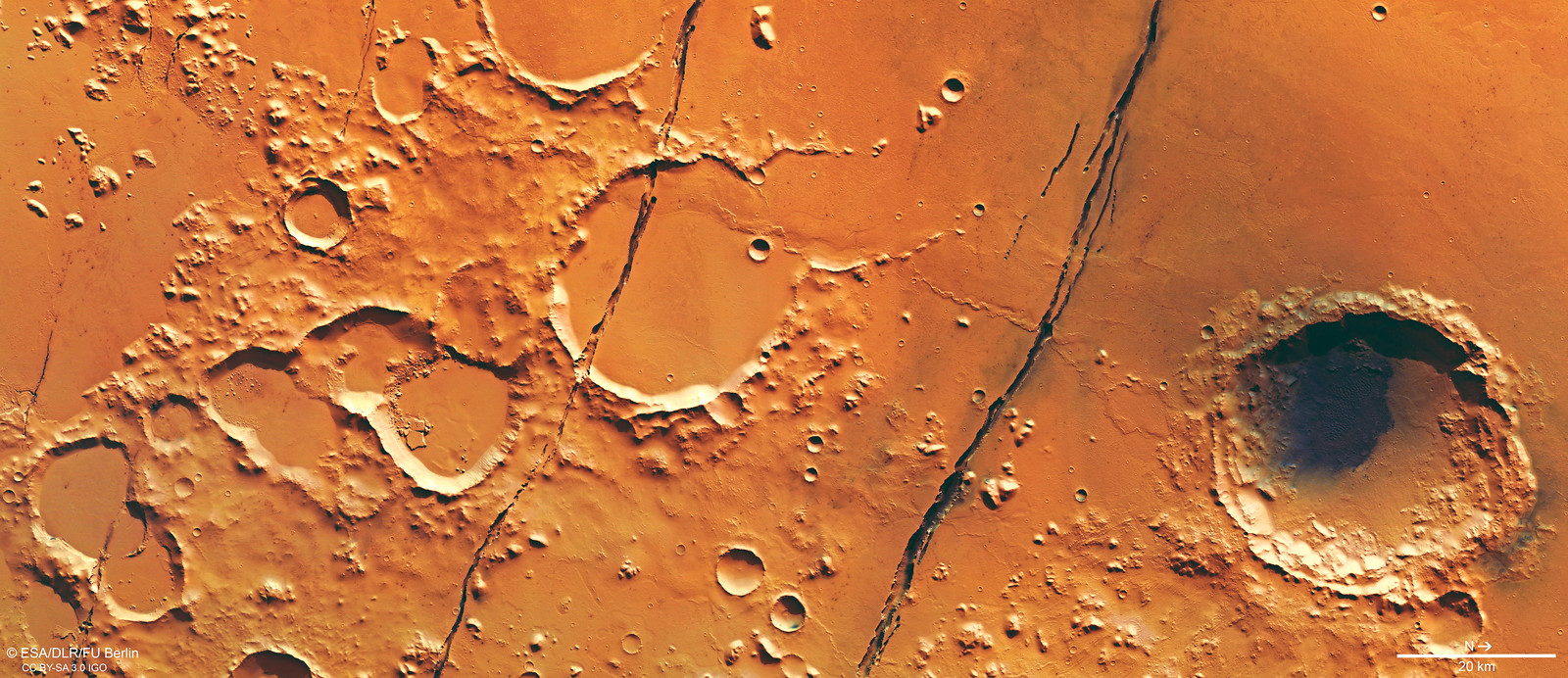This close-up photograph captures the strikingly textured, amber-toned surface of what resembles the planet Mars, characterized by its red, orangey hue. Dominating the right side of the image is a large crater with a notably dark center, suggestive of material that has settled deeper within it. Scattered across the rest of the surface are numerous craters of varying sizes and shapes, including oblong and nearly perfect circular ones, hinting at different impacts and erosions over time. In addition to the craters, the image shows distinct vertical cracks running from top to bottom, especially two prominent ones that stand out in the center, with additional smaller ones to the left-hand side. Further adding to the rugged terrain are numerous small bumps that could be interpreted as tiny mountains or surface irregularities. The lower left corner is marked with the text "E-S-A-T-L-R-F-U Berlin," grounding the photograph in a specific context or study. This combination of features—craters, crevices, and cracks—paints a vivid picture of a once-agitated, now serene planetary landscape.